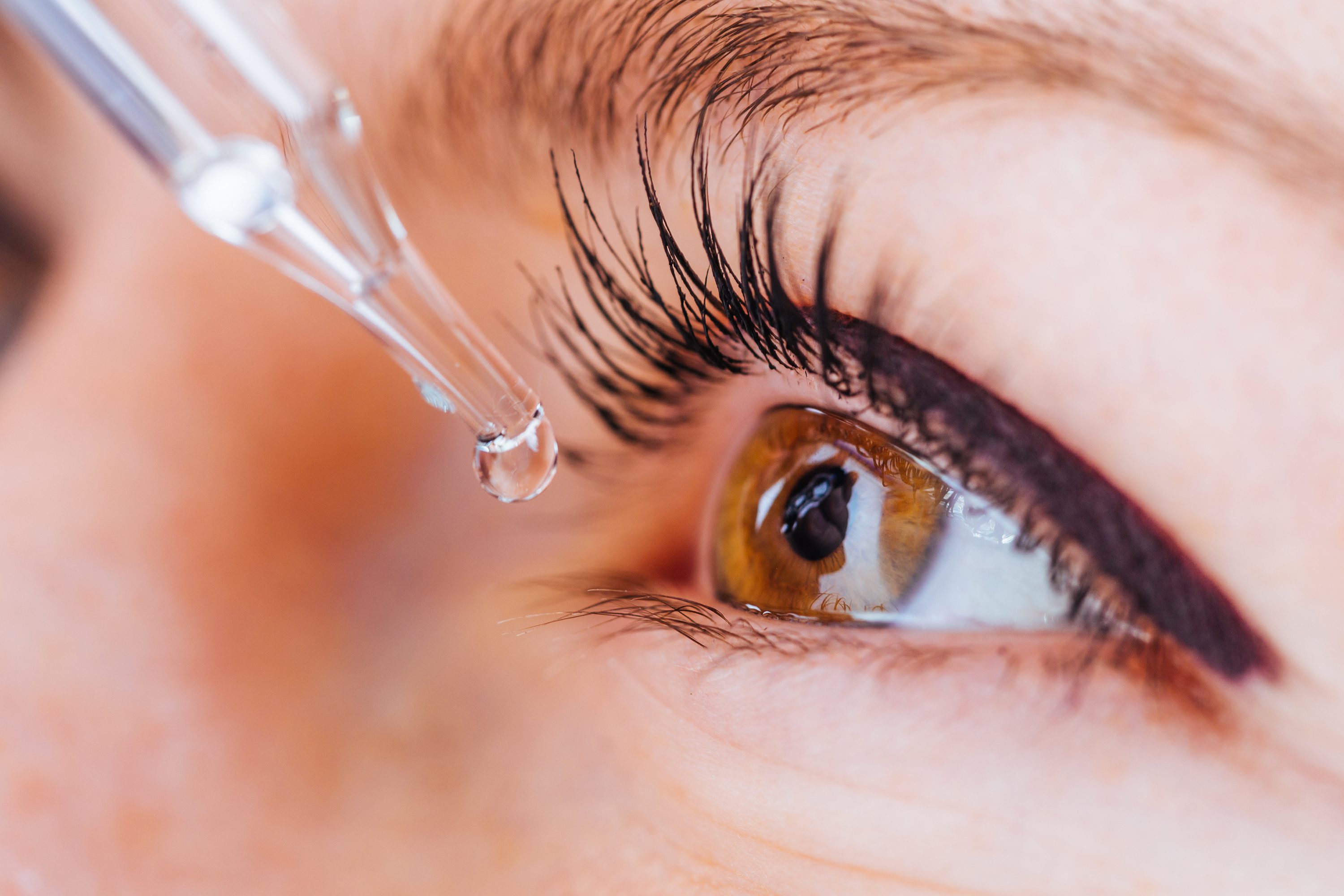In this horizontal, close-up color photograph, a Caucasian woman’s hazel eye is prominently featured in the center of the frame, wide open and staring intently at a clear glass dropper hovering above. The dropper is about to release a transparent droplet of liquid into her eye. Her bold black eyelashes and well-defined brown and black eyebrows accentuate her striking eye, which also has a slightly teary appearance, suggesting the imminent delivery of the eyedrop. There's a hint of pinkish pigment around the eye, contrasting with her fair skin. The detailed image captures the precise moment before the drop settles into her eye, highlighting the delicate act of applying eye drops.